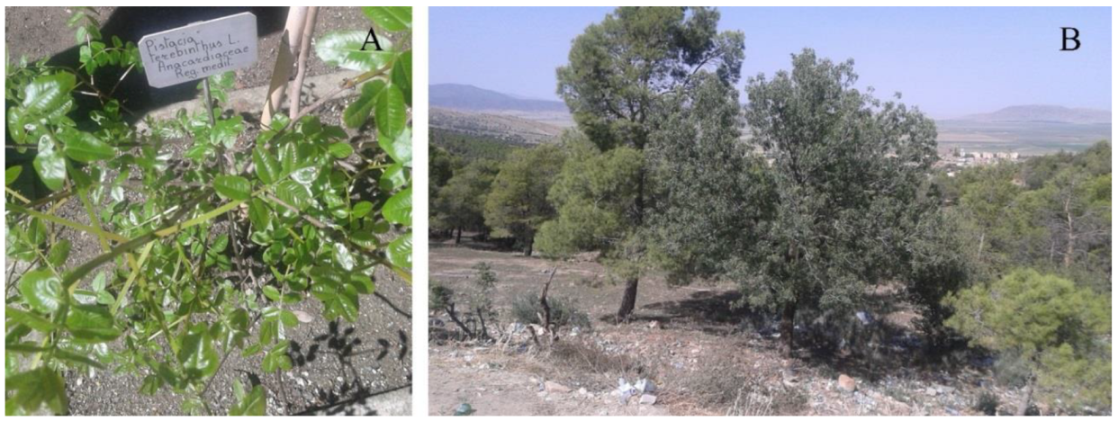The image is divided into two distinct photographs, each identified with the letters 'A' on the left and 'B' on the right, marked in the top right corners. Photo A is a close-up of a very small, vibrant green plant with a white handwritten label on a stake embedded in the soil. The label appears to read "Pistisia," although the handwriting is difficult to decipher. Shadows, possibly from the photographer, fall across the plant. In contrast, Photo B showcases a landscape scene featuring two mature trees standing on a rocky, dirt-covered hill. The foreground is sparse, with primarily white rock and brown dirt, devoid of lush vegetation. Behind these trees lies a valley, further backed by a dense array of additional trees, leading up to a distant mountain range. The sky above is clear blue, and city buildings are faintly visible in the far distance. This dual photograph composition suggests an ecological study area, comparing the growth of different plants in their respective environments.